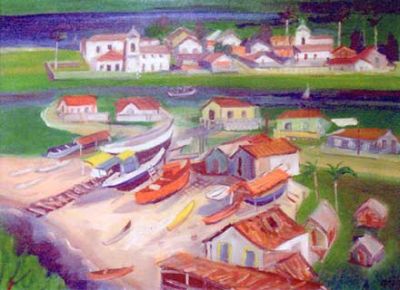This artwork depicts a vivid and densely packed shipyard scene along a layered coastal town. In the foreground, an assortment of small boats, including canoes, kayaks, and fishing vessels, rest on a sandy stretch beside white and red-roofed boat houses and huts, scattered randomly amidst patches of grass and palm trees. To the left, the scene transitions into a grassy area dotted with a mixture of houses and a few larger boats. About two-thirds into the image, a river runs horizontally across, hosting several boats, while behind it, a densely packed town emerges, filled with buildings and perhaps churches with recognizable steeples. Another river is visible towards the top of the image, accompanied by yet more buildings. The entire composition boasts a soft and subtle color palette of whites, oranges, browns, blues, and greens, emphasizing a serene yet bustling coastal atmosphere.